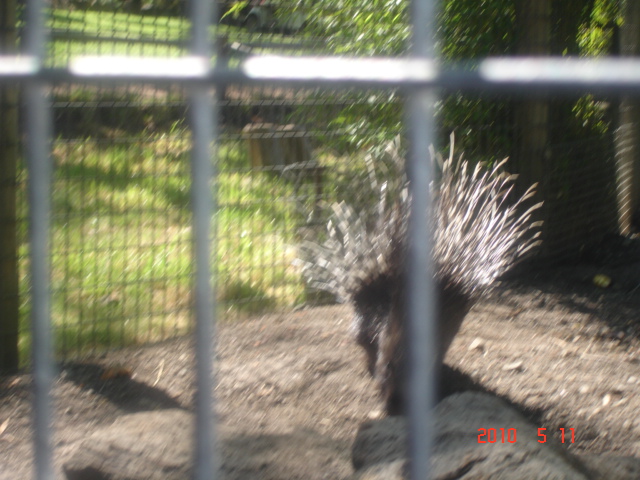This photo captures a somewhat blurry image of an animal enclosure, possibly at a zoo, taken through a metal fence. The enclosure features a ground covered in soil and rock, while the area outside the cage shows grass, vegetation, and trees. The animal inside, though difficult to discern clearly, resembles a porcupine with long needles fanning upward on its back. The bars of the cage are visible in the foreground and bear several red text timestamps. The bottom right corner of the photograph indicates the date 2010-5-11.